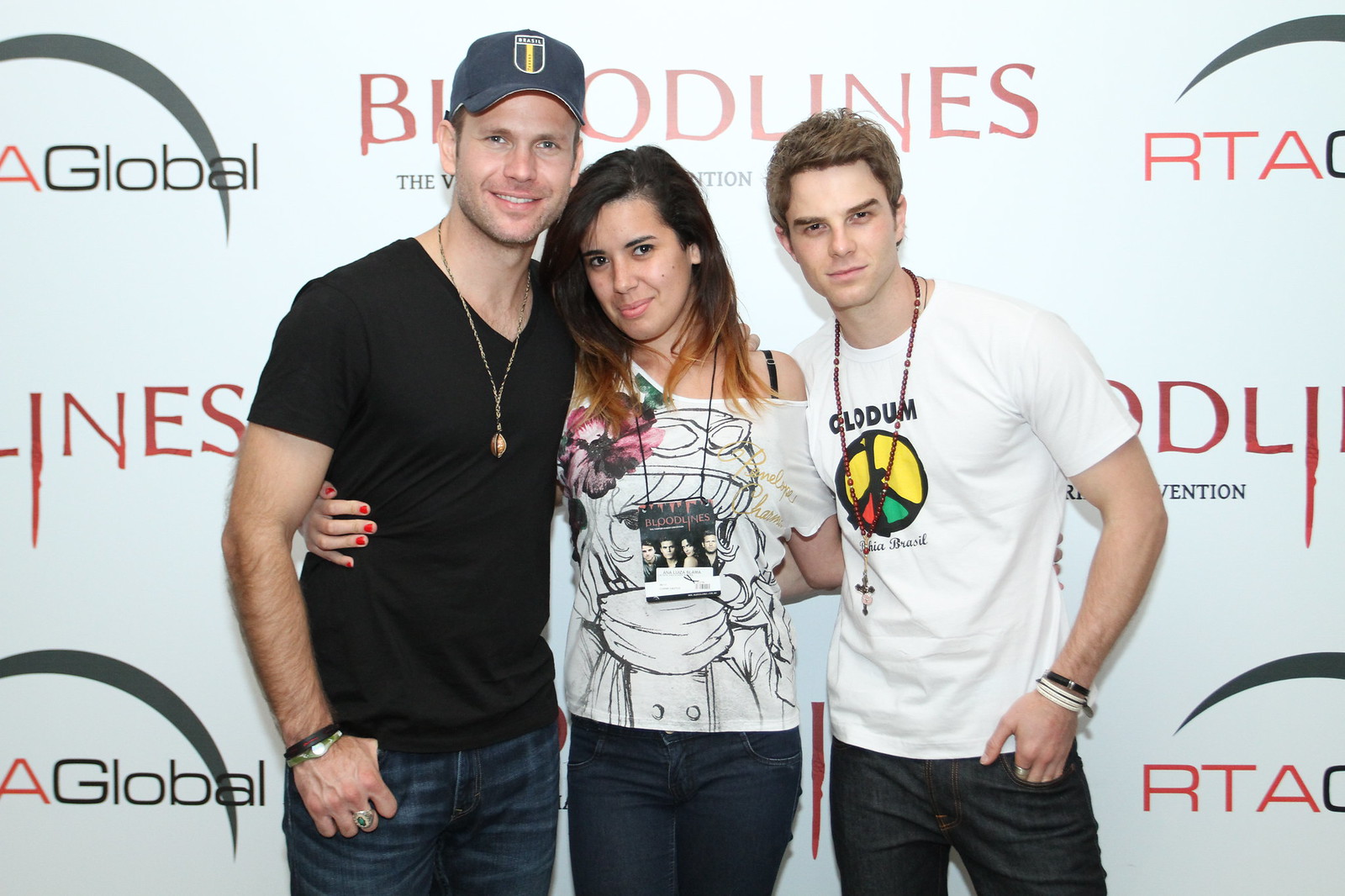In the image, three individuals pose closely together, arms around each other’s waists, in front of a backdrop that reads "Bloodlines" and "RTA Global" in red and black text, suggesting a TV show or convention setting. On the left stands a tall young man, around 5'10", wearing a blue cap, black t-shirt, blue jeans, necklace, and wristbands. He is smiling and looking directly at the camera. In the middle, there is a young woman with dark brown hair and highlighted tips, dressed in a white t-shirt featuring black graphics and dark pants. She’s leaning on the man to her left and smiling brightly. On the right, another young man of similar height, with short, highlighted brown hair, dons a white t-shirt and dark pants. He stands with his fingers in his pockets, also sporting wristbands and a necklace, and is smiling alongside the others. Their casual yet cheery demeanor, combined with the themed backdrop, hints at a fan convention or promotional event.